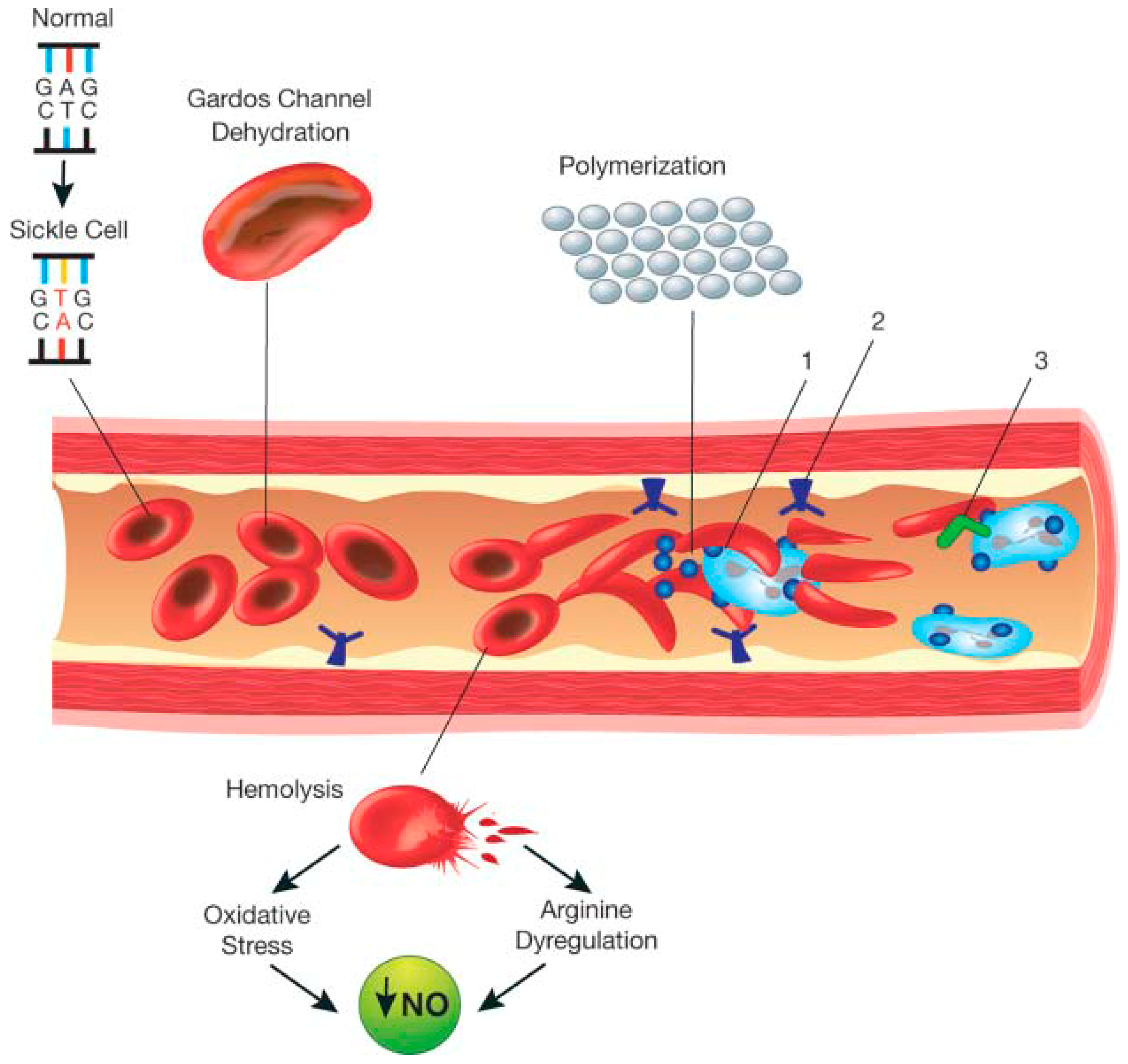This highly detailed and colorful scientific illustration depicts the various effects of sickle cell anemia on blood cells and bodily functions. At the top left, we see the text "normal," accompanied by the genetic sequences G-A-G-C-T-C, signifying typical hemoglobin. In contrast, the section labeled "sickle cell" displays the sequences G-T-G-C-A-C. The image highlights an artery and outlines several pathological processes in sickle cell anemia. 

On the left, a structure labeled "gardos channel dehydration" shows how cells lose hydration. Moving right, "polymerization" is depicted with white ovals, illustrating the formation of rigid polymer structures in red blood cells. Just below, the image points out "hemolysis," indicating the destruction of red blood cells. 

Further annotations include "oxidative stress," and a section pointing toward "arginine deregulation" indicated by an arrow and a green circle labeled "NO" (Nitric Oxide), illustrating the biochemical disruptions occurring within the cells. The image is richly colored in blue, red, pink, green, and black, making it visually engaging while demonstrating the complex and debilitating effects of sickle cell anemia.